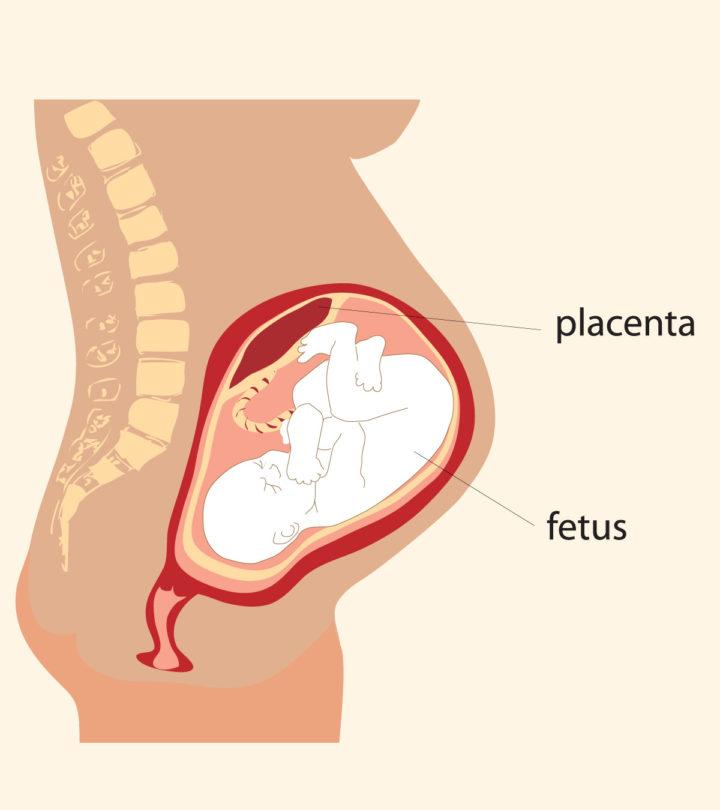The illustration depicts a cartoonish, animated diagram of a pregnant woman from the torso down to the thighs, set against a light pink background. The woman's body is colored in a flesh-tone hue, with her legs appearing slightly more tan. The image provides an inside view of her womb, clearly showing a more detailed white fetus positioned upside down, as if nearing birth. The baby's position is encased in a reddish, pear-shaped outline representing the womb. Labels in black text identify key parts of the diagram: one label points to the "fetus" and another points to the "placenta." Additionally, a basic outline of the woman's spine and some objects behind it are visible, contributing to the medical feel of the image.